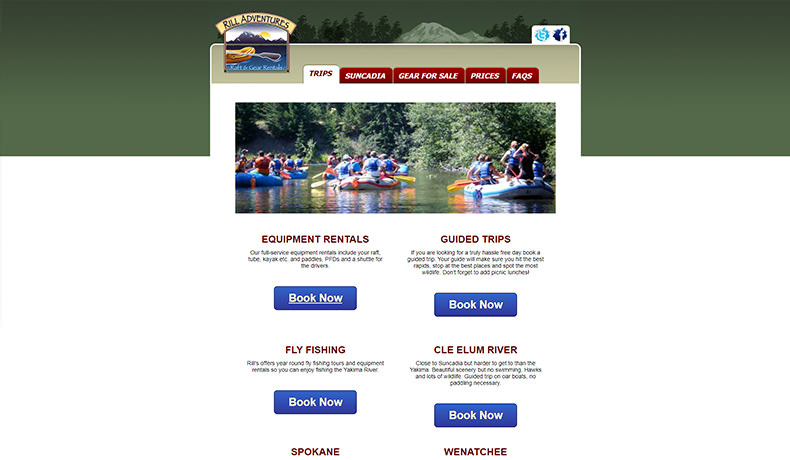The image depicts a website designed for equipment rentals named "Rural Adventures." The layout features a vivid green navigation bar spanning the top, prominently showcasing the company's logo against a picturesque background of towering trees and majestic mountains. The navigation bar includes five tabs, with “Trips” highlighted in white, and the remaining tabs—"Acadia," "Gear For Sale," "Prices," and "FAQs"—displayed in red.

Beneath the navigation bar, there's an engaging image of groups paddling rafts down a river, perfectly capturing the adventurous spirit of the site. Below this captivating photograph, the webpage is organized into four sections arranged in two columns. These sections are titled "Equipment Rentals," "Guided Trips," "Fly Fishing," and "Clay Elam River." Each section provides specific details and is equipped with a blue "Book Now" button, inviting visitors to take immediate action and plan their next rural adventure.